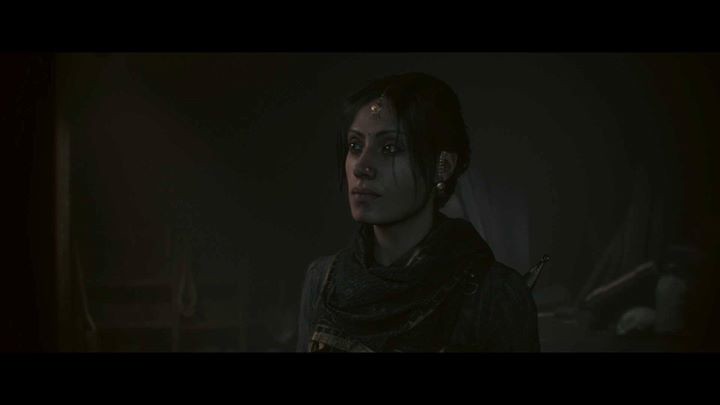The image is a dark, black-and-white still shot, likely from a video game, depicting a woman standing in what appears to be a cave repurposed as living quarters. She is centrally positioned, gazing to the left with realistic features for a digital creation. She has dark, pulled-up hair, gold earrings, and a nose ring. A dark scarf wraps around her neck, complementing her dark jacket or shirt. Notably, she has a symbol resembling a third eye medallion on her forehead, just under her hairline. The blurred and pixelated background includes indistinct items: rocks, perhaps bags of supplies, wooden shelves, a rope, a chair, a jar, and a piece of wood, enhancing the mysterious atmosphere of the scene.